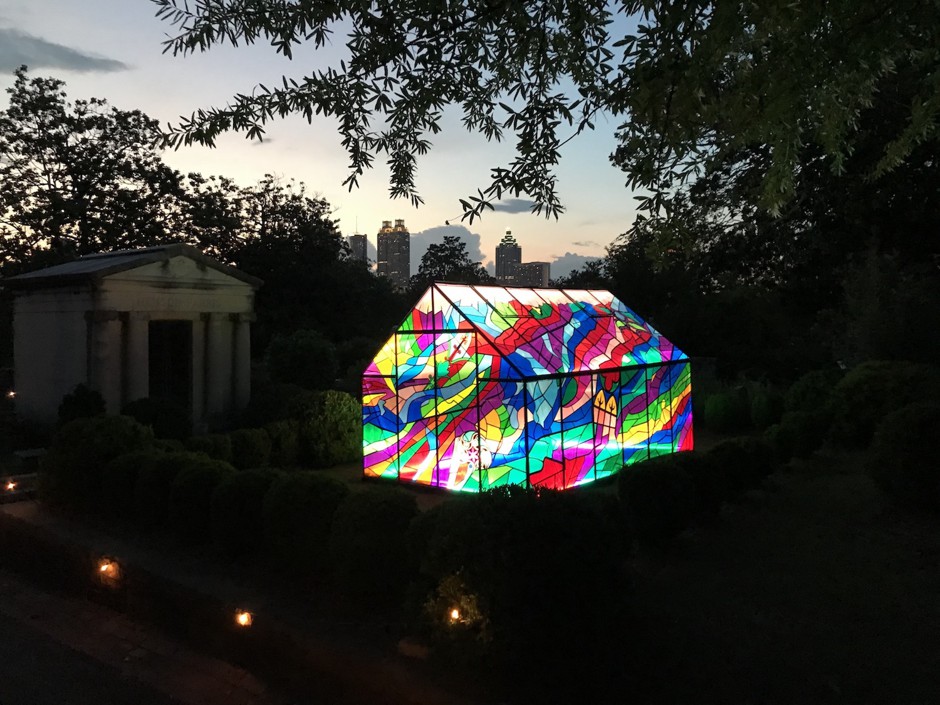This photograph, captured outdoors at the cusp of nighttime, showcases a magical scene in a garden with a cityscape in the background. As the sky transitions from day to night, the lingering glow of the sunset casts a faint light over the clouds and reveals five distant skyscrapers. The primary focus of the image is a vibrant stained glass tent or greenhouse situated in the center. This structure is brilliantly illuminated from within, casting an array of colors, including red, pink, purple, blue, lime green, and bright yellow, in various patterns. It features two doors and a roof with an intricate design. To the left, a small mausoleum or stone shed, made of gray and black concrete, stands quietly amidst the dark silhouettes of leafy trees. The foreground is adorned with a well-manicured grassy area, dotted with lit lanterns along a meandering walkway, enhancing the enchanting atmosphere of the scene.